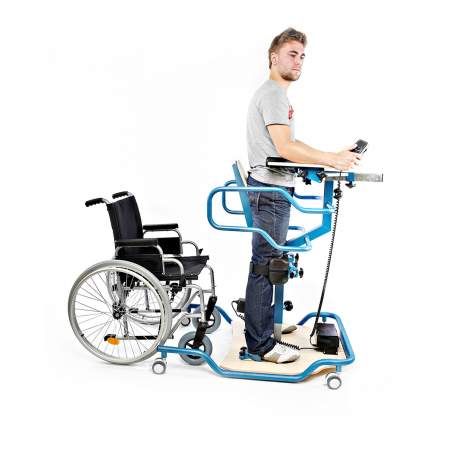In the image, set against a solid white background, two central objects and a man are featured, suggesting a medical or rehabilitative setting. On the left side, positioned toward the bottom, is a side-turned wheelchair devoid of an occupant. The wheelchair is black with gray wheels and appears to be integrated into a unique mobility device. This device includes a blue metal piping bar extending from one side of the wheelchair to the other, supporting the structure at the lower wheels with small gray and white caster wheels. 

On the right side of the image, in front of the wheelchair, stands a man clad in a t-shirt, jeans, and shoes. He is utilizing the mobility device, which seems to function as a support system designed to help individuals who are disabled to stand upright. The man is standing on a small platform and has black braces affixed to his legs. A blue apparatus presses against his back, while he leans forward into a sternum support that wraps around his stomach. In his hands, he holds objects resembling controllers. This detailed setup suggests the device is likely motorized, enabling the user to maintain a standing position for improved mobility, potentially in a clinical or rehabilitation environment.